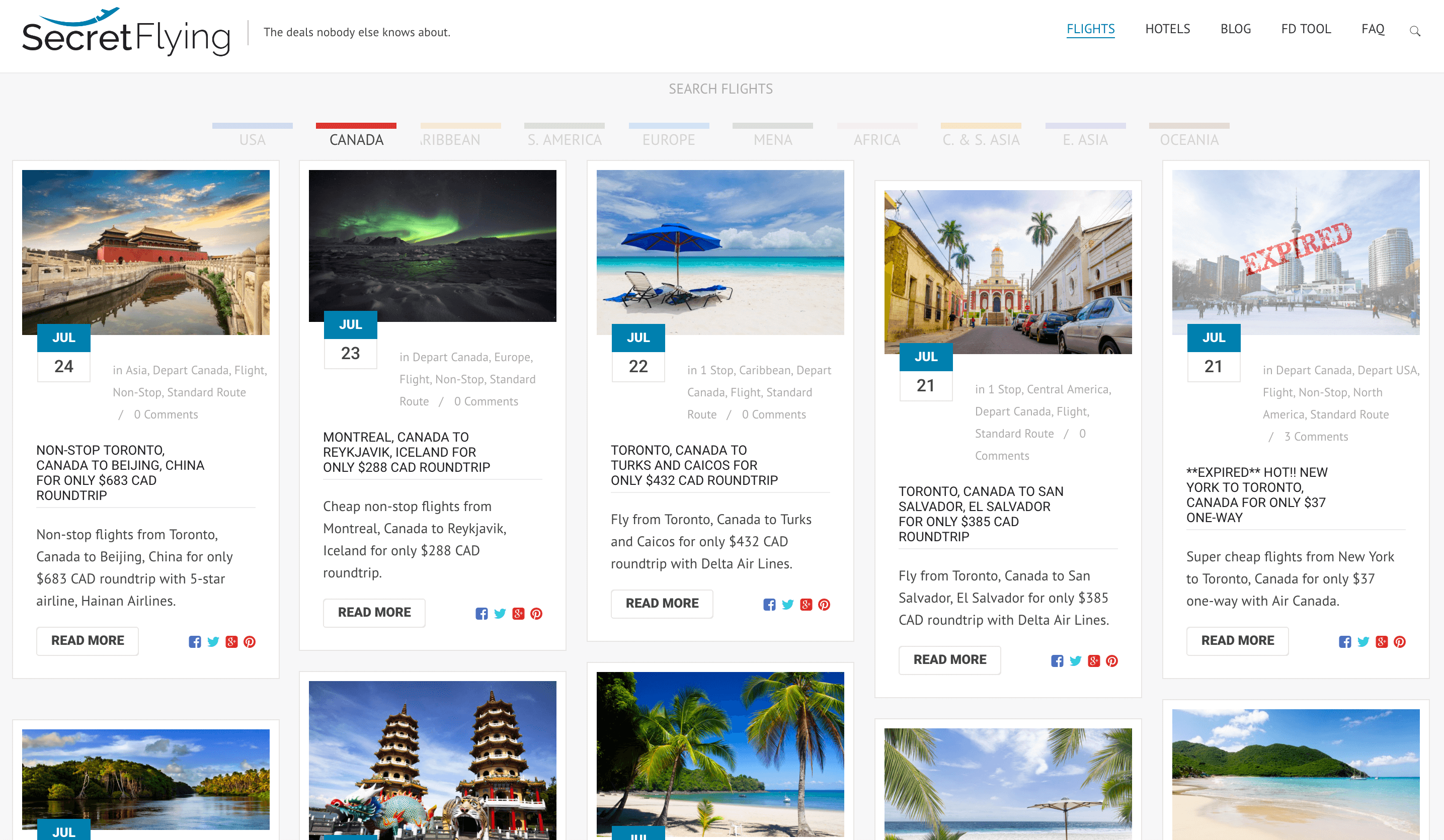The image is a screenshot of the website "Secret Flying," which touts itself as offering exclusive travel deals. The website header includes navigation options such as Flights, Hotels, Blog, FD Tool, FAQs, and a search icon symbolized by a magnifying glass.

The "Flights" section is active in the screenshot, featuring search criteria for booking flights. Users can select departure locations from regions such as the USA, Canada, the Caribbean, South America, Europe, MENA (Middle East and North Africa), Africa, Central and Southern Asia, East Asia, and Oceania.

Several flight deals are listed, including:
- A non-stop flight from Toronto to Beijing in July.
- A flight from Montreal to Reykjavik, Iceland, on July 23.
- A flight from Toronto, Canada, to Turks and Caicos.
- A flight from Toronto to San Salvador, El Salvador, on July 21 for only CAD 385.
- A New York to Toronto one-way flight for only USD 37, although this deal has expired as of July 21.

The website highlights that it offers significant travel savings, but potential buyers need to act quickly to secure these deals.